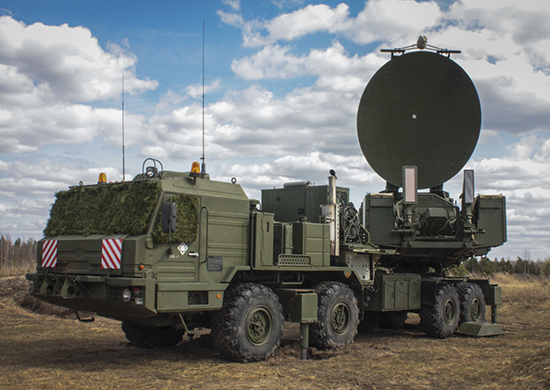This image showcases a robust military-style truck parked on a flat, patchy dirt field with yellowish-brown grass and sparse green foliage in the background under a clear blue sky with scattered white clouds. The truck, entirely olive green with black and forest green-rimmed tires, features a distinctive cube-shaped front adorned with red and white warning stripes on either side of the grille. Orange lights are mounted atop and along the vehicle's sides, and black antennas extend from either side. Green camouflage material or moss is draped over the windshield, obscuring the view inside. 

The truck is segmented into two parts: the main body with a short bed carrying various equipment, and an attached trailer. The trailer has large tires and supports a platform that angles upward, bearing a prominent, giant green circular structure, likely a radar or satellite dish. Overall, this heavy-duty vehicle, equipped with specialized military hardware, appears designed for reconnaissance or communication tasks.